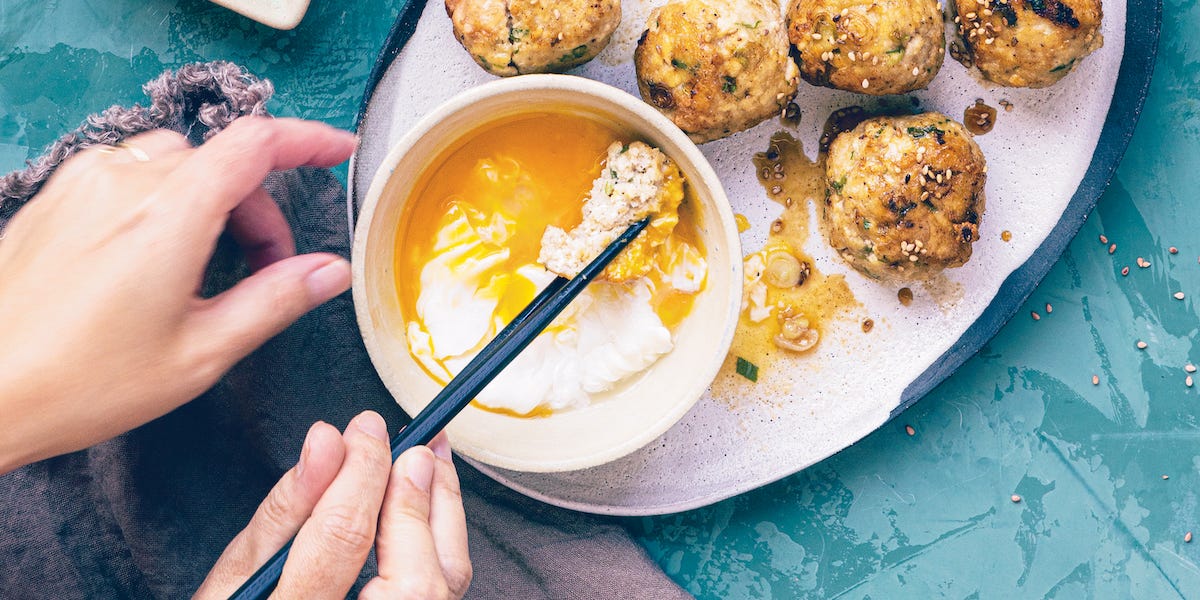In this photograph, we observe a close-up view of someone eating at a table with a bluish marble-like surface, blending light and dark blue tones. The table is set with a light gray napkin positioned to the left, upon which the person's left hand rests. Their right hand, holding a pair of dark blue chopsticks, is dipping food into a small white bowl containing a partially cooked egg with a runny yolk.

The primary dish on the table is presented on an oval white plate with a dark blue rim. It features several small, round, brownish items that resemble meatballs or dumplings, sprinkled with sesame seeds. The hands visible in the image, which appear to be female, are unadorned with nail polish. The composition of the photograph gives a feeling of intimacy, as if you were looking down at your own meal. The overall setup, the chopsticks, and the meatball-like food suggest an Asian cuisine setting.